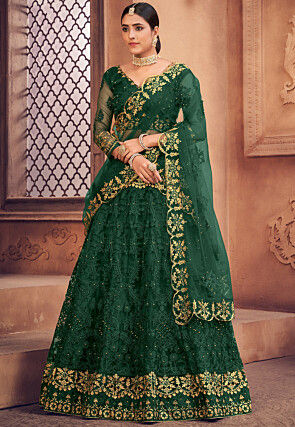The photograph features a young Indian woman standing gracefully in a sophisticated, traditional green dress adorned with intricate yellow/gold embroidery along the bottom, the edges of the sleeves, and a decorative sash across her chest. The elegant attire includes super long sleeves that extend beyond her knees. Her black hair is neatly parted in the center and pulled back into a ponytail, accentuated by a distinctive piece of gold jewelry where her hair is parted at the center. She also wears a striking array of jewelry including a white beaded choker necklace, matching earrings, and large silver bracelets or bangles on her wrists, along with several prominent rings on her fingers. She stands with her hands in front of her, looking slightly to the left of the image. The backdrop features a beige-colored wall with a large window and some inclined steps, contributing to the overall elegance and traditional charm of the scene.